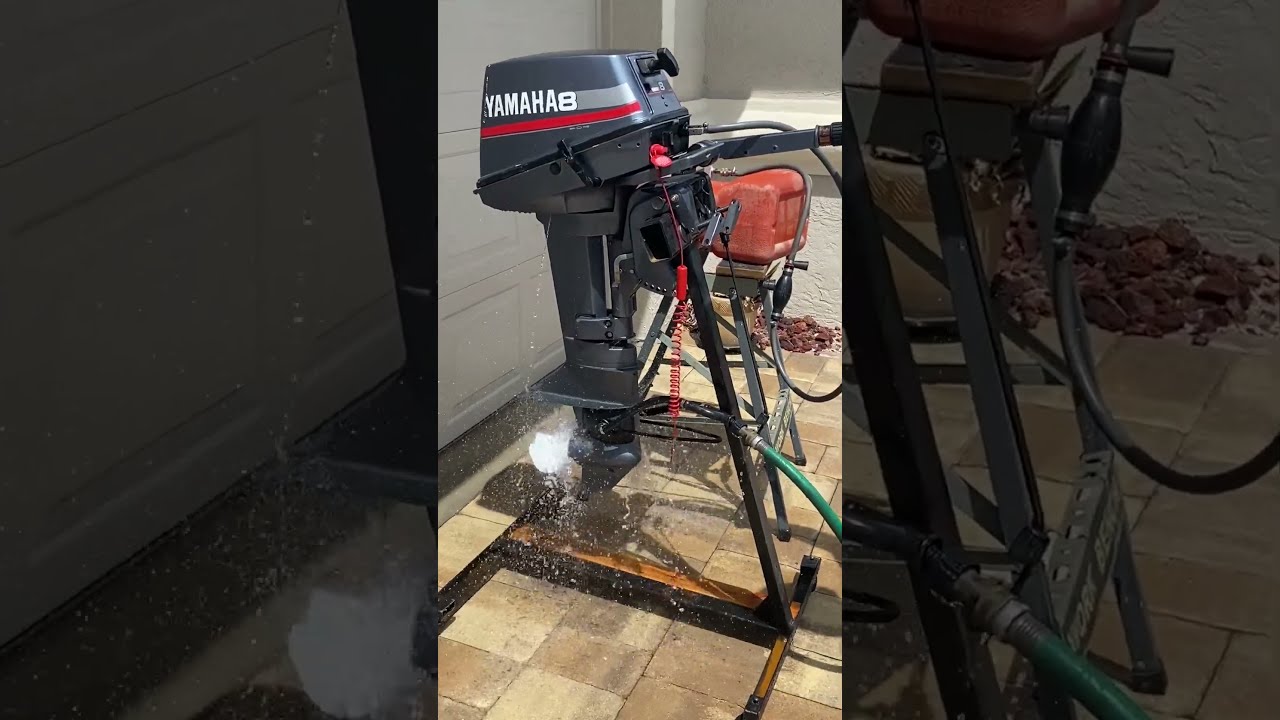The image shows an older Yamaha 8 horsepower outboard boat motor, predominantly gray with white "Yamaha" lettering at the top. Below the branding, there is a red stripe accented by a black pull handle. The motor is mounted on a stand on a tile patio outside, which appears to be in front of a beige garage door, illuminated by daylight. Attached to the motor is a black hose, likely used for cooling the engine during testing. In the background, there is a 5-gallon gas container lying on its side, accompanied by various tubing and possibly a water hose. Water seems to be spewing from the engine, indicating that it is running, with the propeller possibly spinning.